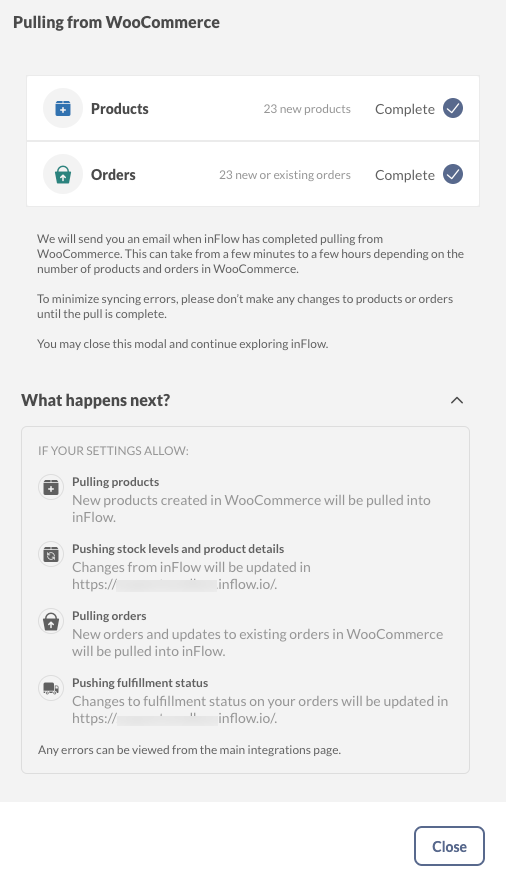Screenshot in Portrait Orientation Detailing WooCommerce Data Sync Process

The screenshot is in portrait orientation with a pale grey background, transitioning to white at the bottom. In the bottom right corner, a dark blue button with rounded corners reads "Close."

At the top left, bold black text states: "Pulling from WooCommerce.” Below this, a white rectangular section spans the screen, containing two entries in bold text: "Products" and "Orders."

- **Products**: Accompanied by a blue file folder icon, it states "23 new products" in small text, with a blue circle check mark indicating completion.
- **Orders**: Paired with a green shopping basket icon, it notes "23 new or existing orders" in small text, also marked complete with a blue circle check mark.

A thin line separates the "Products" and "Orders" sections.

Returning to the grey background for the remainder of the page, small text explains the syncing process: 

"We will send you an email when InFlow has completed pulling from WooCommerce. This can take from a few minutes to a few hours depending on the number of products and orders in WooCommerce. To minimize syncing errors please don't make any changes to products or orders until the pull is complete."

The section concludes with a heading, "What Happens Next," followed by a list detailing the subsequent steps.